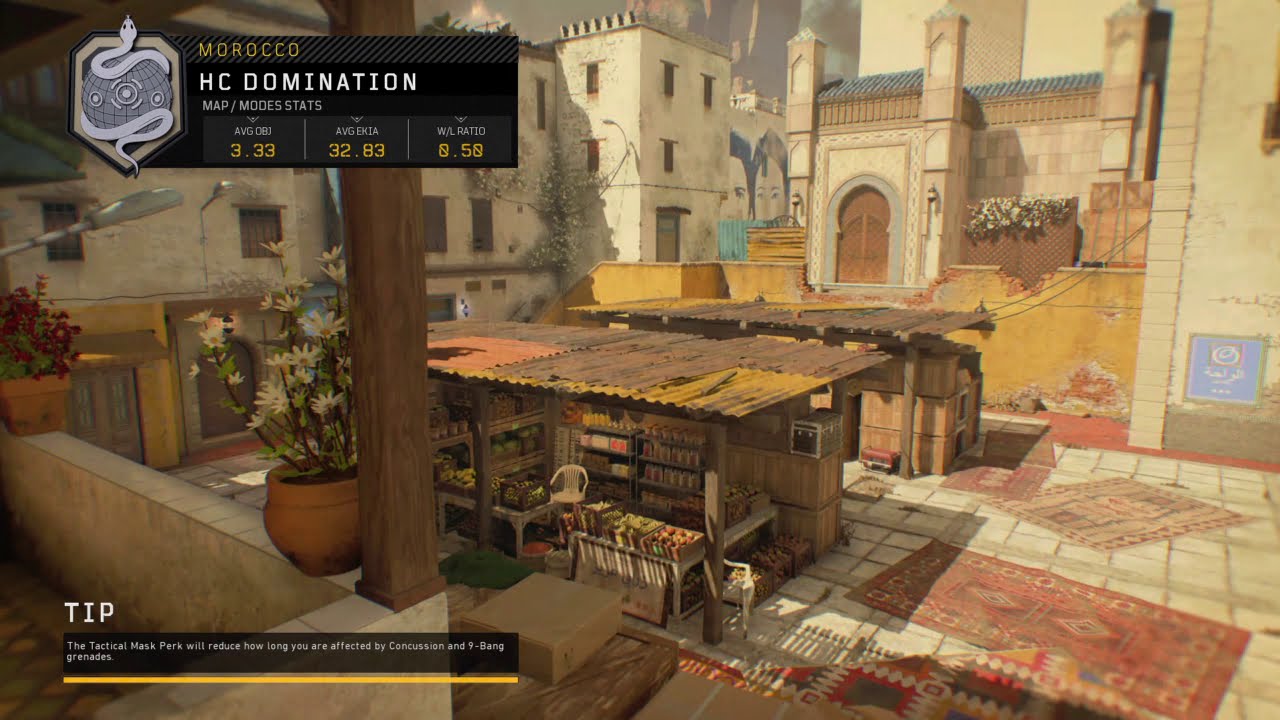The image is a highly detailed screenshot from a video game, specifically a map called "Morocco HC Domination," as indicated by a black box in the top left-hand corner. This box displays a shield symbol with a silver snake wrapped around a dark gray globe, which is adorned with three target-like circles. Below the map name, the text reads "Map/Mode Stats," followed by player statistics, where the first one is "average OBJ 3.33."

The scene itself depicts an intricately designed Moroccan town marketplace, showcasing traditional Moroccan architectural elements. The marketplace is bustling with activity, featuring small market stalls with rusted metal roofs, laden with fruits and various goods. Persian rugs are strewn across the rocky ground, enhancing the authentic feel. The town is surrounded by tall, light-gray stone buildings, which exhibit Arabic influences in their design, including white facades, rounded-top brown doors, and decorative pillars. Pots with colorful flowers and plants add life to the scene, contributing to the vivid portrayal of a traditional Moroccan setting. Towards the bottom of the image, tips on the tactical mask perk are displayed, explaining its functionality in reducing the duration of concussion and 9-bang grenade effects.